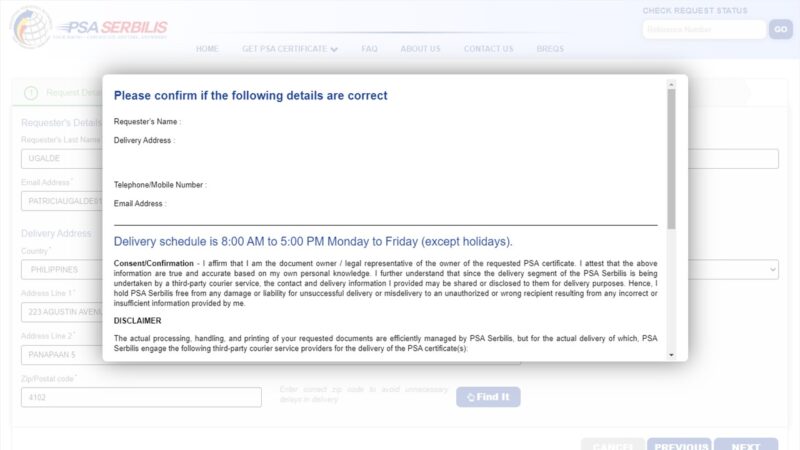This is a detailed screenshot of a computer monitor displaying a website with an active pop-up window in the foreground. The background webpage is heavily faded and hazed over, but visible in the top left corner is a globe-like icon in white, adorned with a blue arrow and a red arrow. To the right of the icon, a bold blue text reads "PSA," and next to it, bold red text says "Surbills." Other small white text is indistinguishable.

Dominating the screen is the central pop-up window with a white background, featuring a vertical gray scroll bar on the far right side. At the top left of this window, a blue heading prompts, "Please confirm if the following details are correct." Below this heading, in black text, are labels: "Requester's Name," "Delivery Address," "Telephone," "Mobile Number," and "Email Address," each followed by the text "nothing entered." 

Beneath a horizontal gray line, blue text states, "Delivery schedule is 8 a.m. to 5 p.m. Monday to Friday except holidays." Following this statement are two paragraphs in black text. The first paragraph is titled "Consent Confirmation" in bold black, and the second, smaller paragraph is labeled "Disclaimer," also in bold black.

At the very bottom lower right-hand corner, at the end of the scroll bar, there is a small gray down arrow.